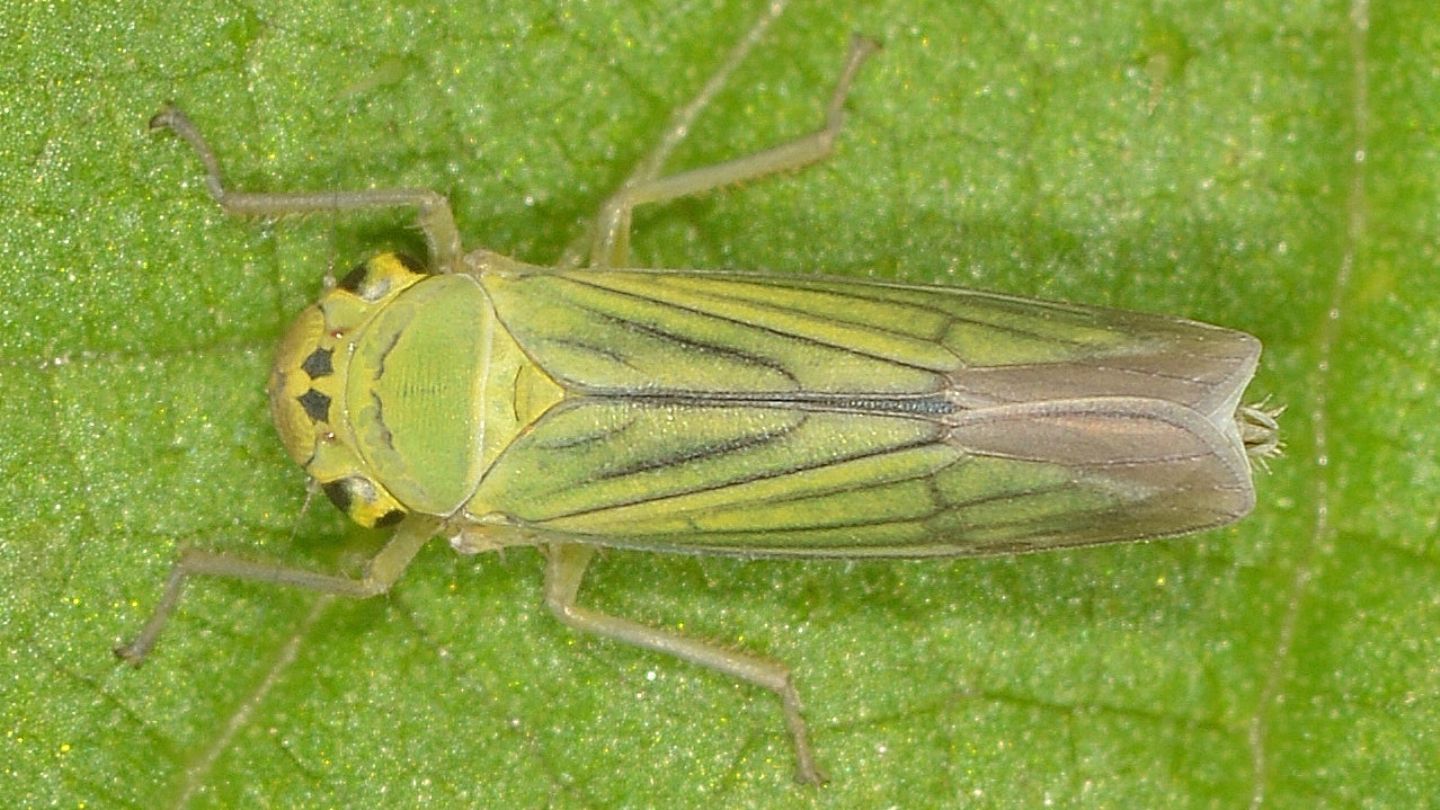This vivid and detailed photorealistic image captures a close-up view of an insect resting on a green leaf, where the intricate veins of the leaf are visible in the background. The insect is centrally positioned, with its head oriented toward the left and its tail to the right. Its body is patterned with striking green and yellow hues, featuring various geometric designs and stripes. The head is a mix of yellow and brown with two wide-set eyes that are black and yellow. The insect has six legs—two of which are antennae pointing forward—and its back legs are bent, giving it a perched stance. The wings are folded over its body, showcasing a predominantly green color that fades into light brown near the tail, adding to its rectangular shape. The overall background is a solid green with a sparkly appearance, enhancing the detailed texture of the leaf.